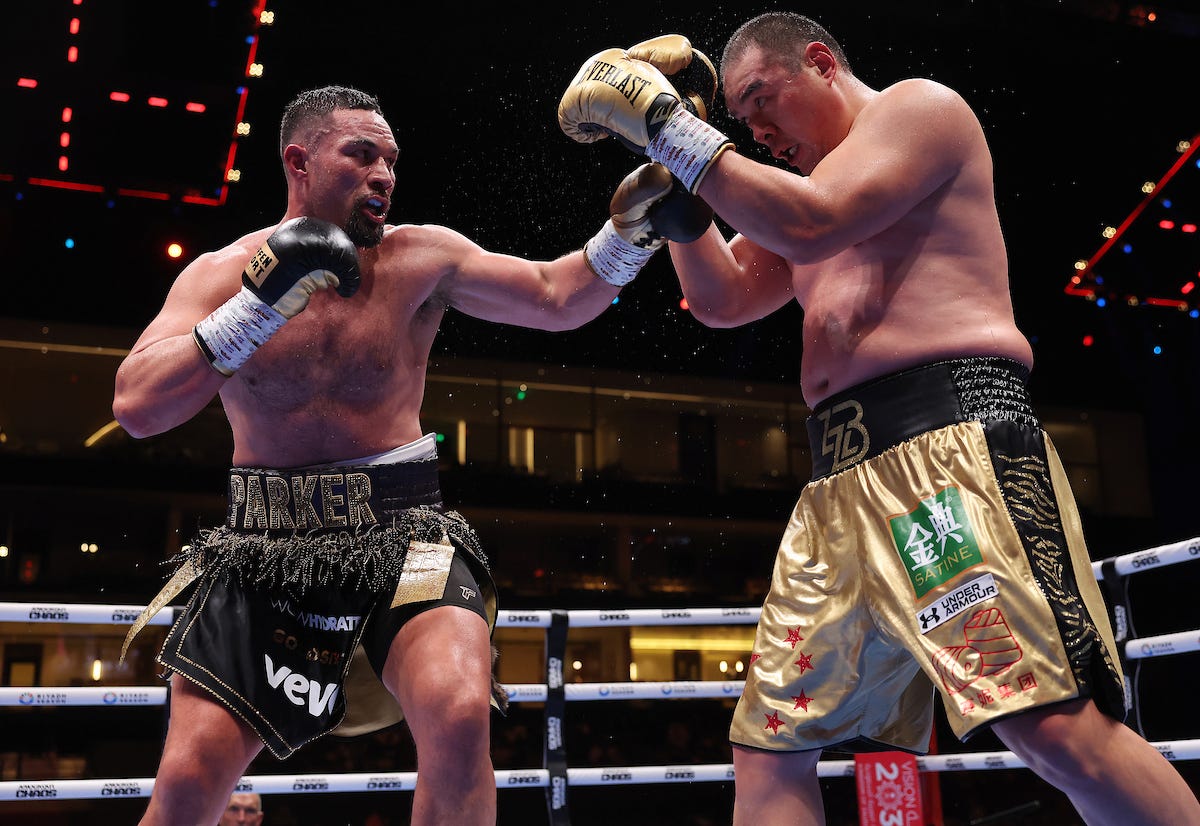In this dynamic, live-action photograph, we see an intense boxing match between two fighters in a dimly lit arena with faint red and blue lights in the background. The fighter on the left, identified by the name "Parker" emblazoned on the waistband of his black trunks, is in mid-action, delivering a powerful punch. Parker's attire includes black boxing gloves and shorts, which appear to have feathers or some other elements dangling from them, and he sports short, cropped dark hair.

Opposite him, the fighter on the right is trying to block Parker's punch. This boxer is outfitted in gold and black trunks adorned with patches, including one from Under Armour and another labeled "Satine" with Asian characters. He wears matching gold Everlast boxing gloves and is heavier, with his belly slightly protruding over his shorts.

The boxing ring features a white canvas and black posts. The surrounding area is dark, obscuring the audience, though a face, possibly of a judge, can be faintly seen focusing on the bout. The fighters are captured in motion, glistening with sweat as they exert all their energy to battle each other fiercely.